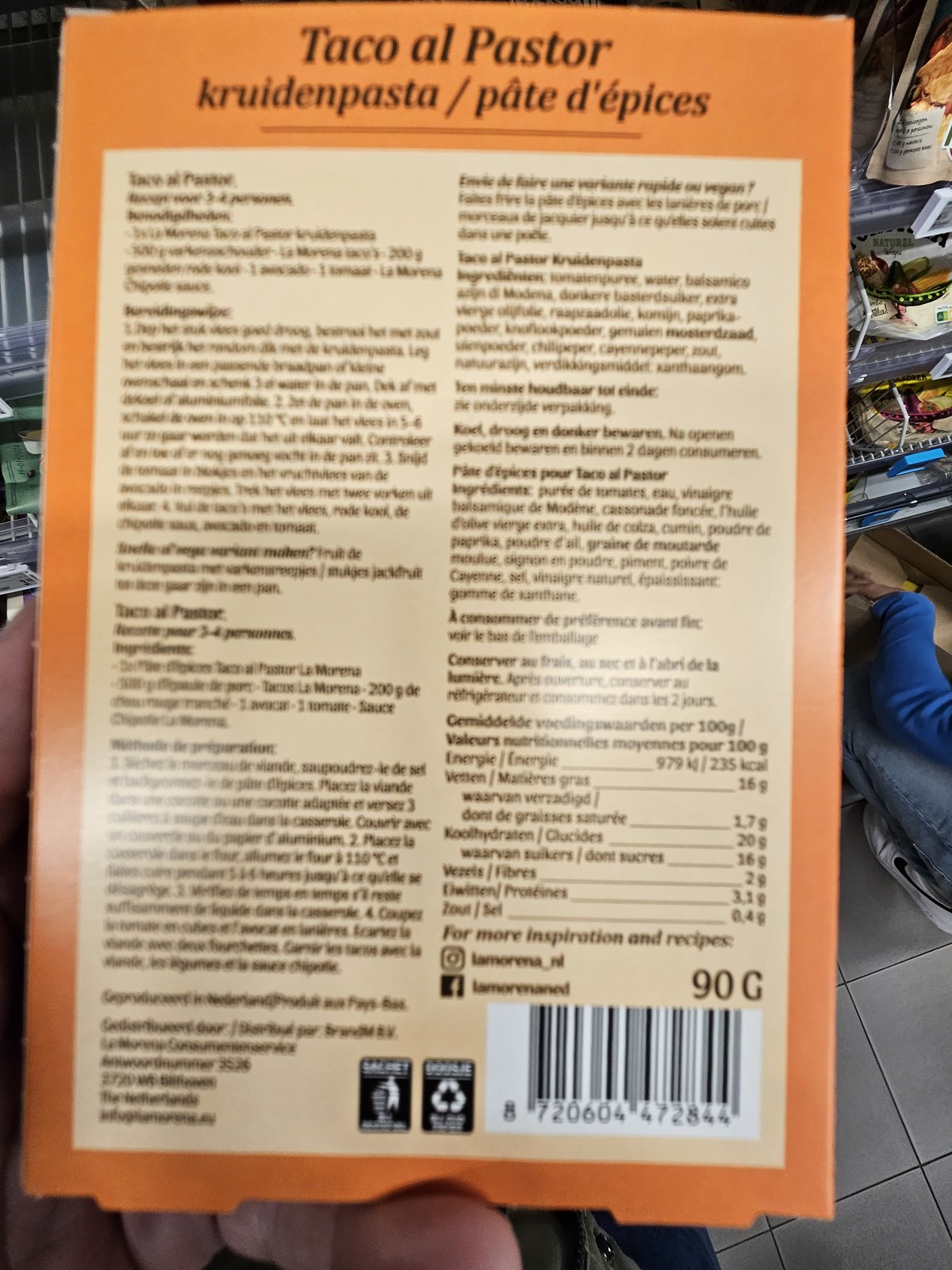A close-up image of the back of a recipe box held by someone's fingers. The recipe featured is for "Taco al Pastor," written in Spanish. Below it, the recipe titles appear in German as "Crudimpasta" and in French as "Pâte d'épices." The box also displays a list of ingredients, a nutrition label, and detailed instructions for making the tacos. In the background, there are shelves with various items, and a person is crouched down, organizing or placing something on the shelves.